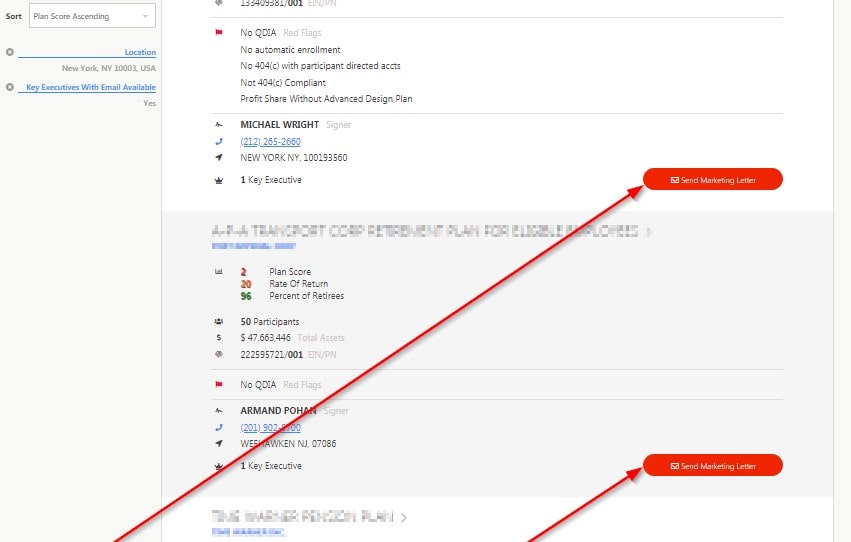This image depicts a detailed view of a web page designed for business analysis and marketing purposes. The layout is structured with a taskbar on the far left-hand side that contains drop-down options labeled "Sort," "Plan," and "Score," with an ascending order preference.

Just below this taskbar, the section begins with a highlighted blue bar displaying the location as "New York, New York, 10003, USA." The page also notes that key executives with emails available are present, marked by the word "Yes" in blue.

On the right-hand side, there are multiple segments separated by bars, containing extensive textual information. The segment mentions “No QDIA red flags,” indicated with a red flag icon to its left. Details such as “No automatic enrollment,” “No 404C with participant-directed accounts,” “No 404C compliant,” and “Profit share without advanced design plan” are listed. Below this section, the name “Michael Wright” appears alongside a blue telephone icon with the phone number 212-265-2660.

Further detailed is another location noted as "New York, New York, 10019-3560" followed by information about a key executive, marked with a crown icon. Within the same box, a red notification states "Send Marketing Letter." Arrows extend from the bottom of the screen, pointing towards red boxes, suggesting a call to action or additional links.

Additional numerical data is presented: a "Plan Score" with an unclear rating, an orange indicator showing "20% of retirees," a green figure of "96," and data about the plan, including "50 participants" and "47,663,446 total assets." An EIN/PN number "22-2595721-001" is also listed. Another red flag icon highlights “No QDIA red flags” followed by the name "Armin Pohan signer" and partially obscured numbers starting with “201-902.” The location "Washahookan, New Jersey, 07086" is mentioned.

Towards the lower right of this detailed view, another red rectangle captioned "Send Marketing Letter" is visible, indicating a repeat call to action. The page is densely packed with key actionable insights and administrative information structured for efficient user navigation.